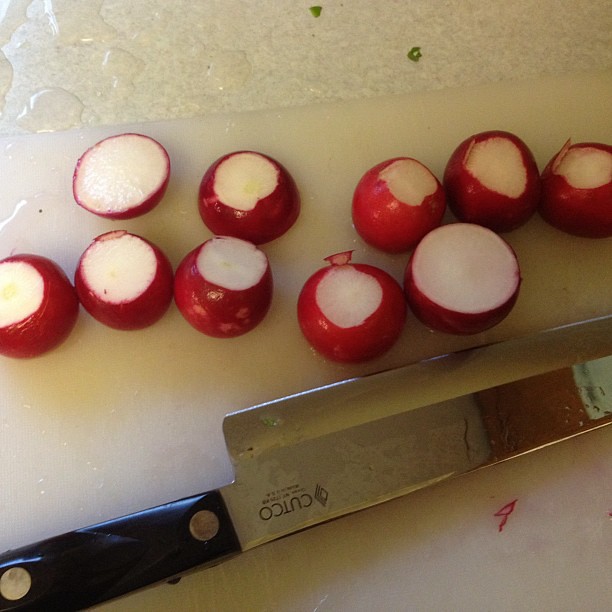The image is a close-up of a vertical, frosted white cutting board on a light gray countertop with some water and small green dots near the top left corner. The cutting board, featuring ten red radishes with their tops sliced off to reveal their white interiors, is arranged in two horizontal rows of five. Some radishes are sliced in half while others remain whole, varying in size. A large, sharp knife with a black handle marked by two silver circles is positioned diagonally from the bottom left, with the blade pointing toward the top right corner. The handle is partially cut off by the edge of the image, and the broad silver blade dominates the middle of the picture. The cutting board is clearly distinguished by its bright, clean appearance contrasting with the surrounding countertop.